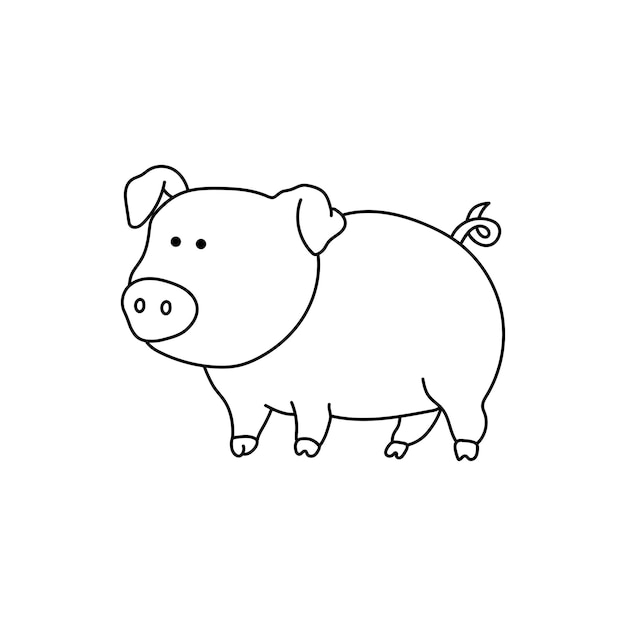This image is a simplistic, amateur black and white hand drawing of a pig. It features a black outline of the pig positioned in profile, facing left. The pig has a round, large body supported by four short legs, each ending in pointed hooves. Its head displays two small, black circular eyes and a prominent snout with two nostrils depicted as hollow circles. The pig's ears fold forward from the top of its head, and a short, curly tail is visible at its rear. The drawing is devoid of any color, shading, or additional details, making it look like a basic sketch possibly created with a pen or pencil, or perhaps using a simple digital tool like Microsoft Paint. It stands alone on a white background without any framing or extraneous elements, giving it a very plain and unfinished appearance.